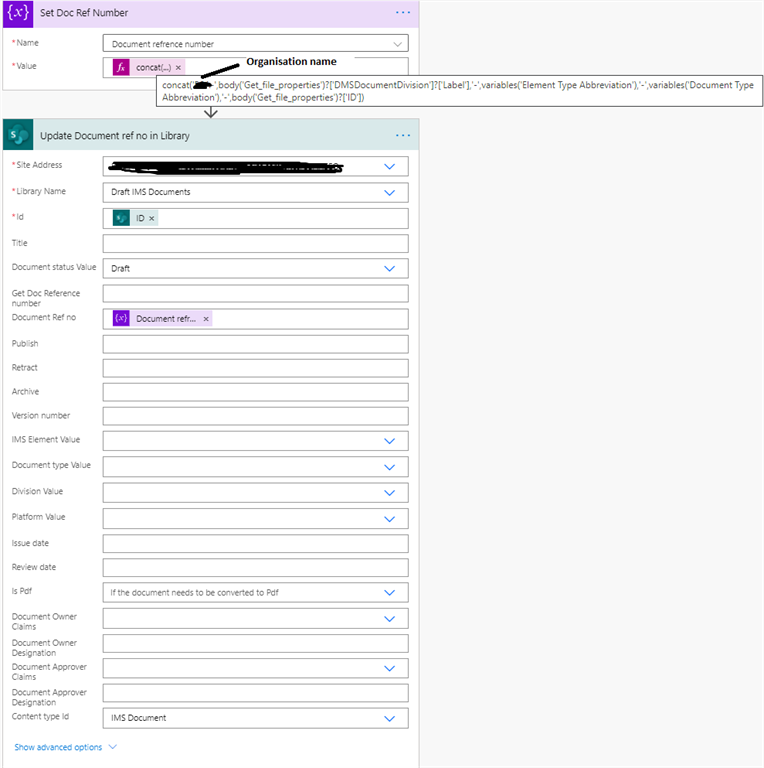The image displays a detailed website interface designed for document management. The top portion features several drop-down menus and input fields, all contained within a user-friendly layout. At the very top, a light purple header banner reads, "Set Doc Ref Number." Below this purple strip lies a white rectangular section labeled "Name" and "Value," each accompanied by a red dot to the left. Beside "Name" is a rectangular drop-down box containing the text "Document Reference Number," while beside "Value" is another box, slightly pink within the white rectangle, with the text "Concat," which is somewhat difficult to read.

Beneath these components, a prominent rectangular text field is labeled "Organization Name," with a connecting black line pointing to it for clarity. 

Following this section is a secondary section separated by a green strip labeled "Update Document Ref No in Library." This section is equipped with numerous drop-down boxes and input fields for detailed document categorization. The fields include "Site Address" (with a red dot beside it and a corresponding drop-down menu), "Library Name" (also marked with a red dot and containing "Draft IMS Documents"), and "ID" (again indicated with a red dot).

Additional fields listed vertically include "Title," "Document Status Value," "Get Doc Reference Number," "Document Ref Number," "Publish," "Retract," "Archive," "Version Number," "IMS Element Value," "Document Type Value," "Division Value," "Platform Value," "Issue Date," "Review Date," "PDF," "Document Owner Claims," "Document Owner Designation," "Document Approver Claims," "Document Approver Designation," and "Content ID." 

Each of these fields is designed to capture specific details through drop-down menus or text input, providing comprehensive document metadata options. 

At the bottom left of the interface, in blue text with a corresponding downward-pointing arrow, it indicates "Show Advanced Options," inviting users to access more detailed settings if needed. The overall layout is highly functional, aimed at effectively managing and categorizing a wide array of document attributes.